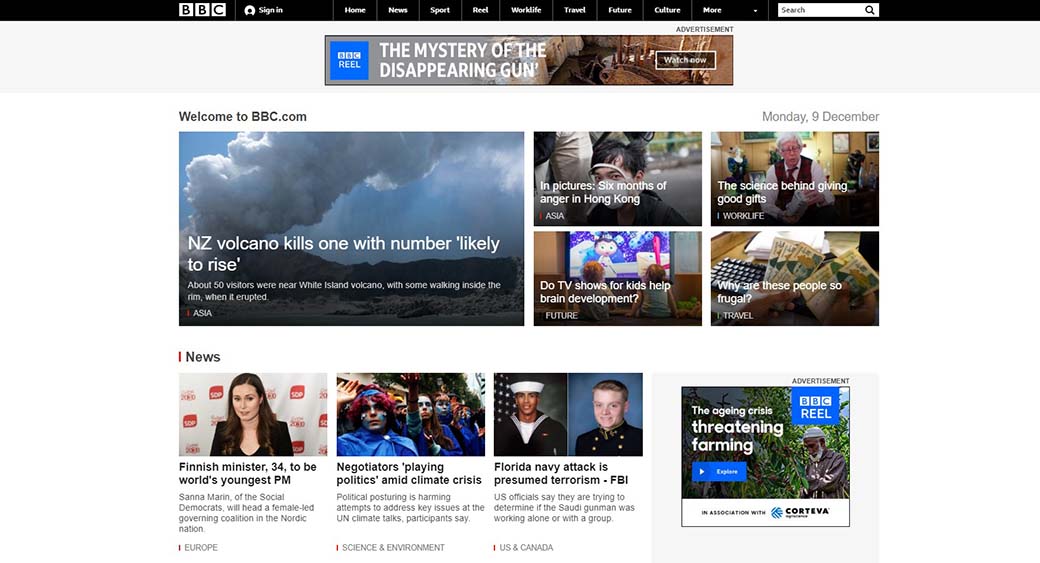The image is a screenshot taken from the BBC website. At the top, "BBC" is prominently displayed with each letter ("B," "B," and "C") in its own separate white box and in bold black font. To the right of the logo, there are navigation links including "Sign in," "Home," "News," "Sport," "Reel," "Worklife," "Travel," "Future," "Culture," "More," and a search bar.

Further down, there is an advertisement with the headline "Worklife" and the title "The Mystery of the Disappearing Gun," accompanied by a "Watch now" prompt, clearly marked as an advertisement.

Below the advertisement, a welcome message reads, "Welcome to BBC.com," followed by a series of news articles with corresponding images. The headlines include:
1. "NZ Volcano Kills One with Number Likely to Rise" - Reporting that about 50 visitors were near the White Island volcano during its eruption, with some even inside the rim; categorized under "Asia."
2. "In Pictures: Six Months of Anger in Hong Kong" - A visual chronicle of the recent unrest in Hong Kong.
3. "The Science Behind Giving Good Gifts" - An article exploring the psychological aspects of gift-giving.

Several other articles are listed below, each paired with relevant images to give a preview of their content.